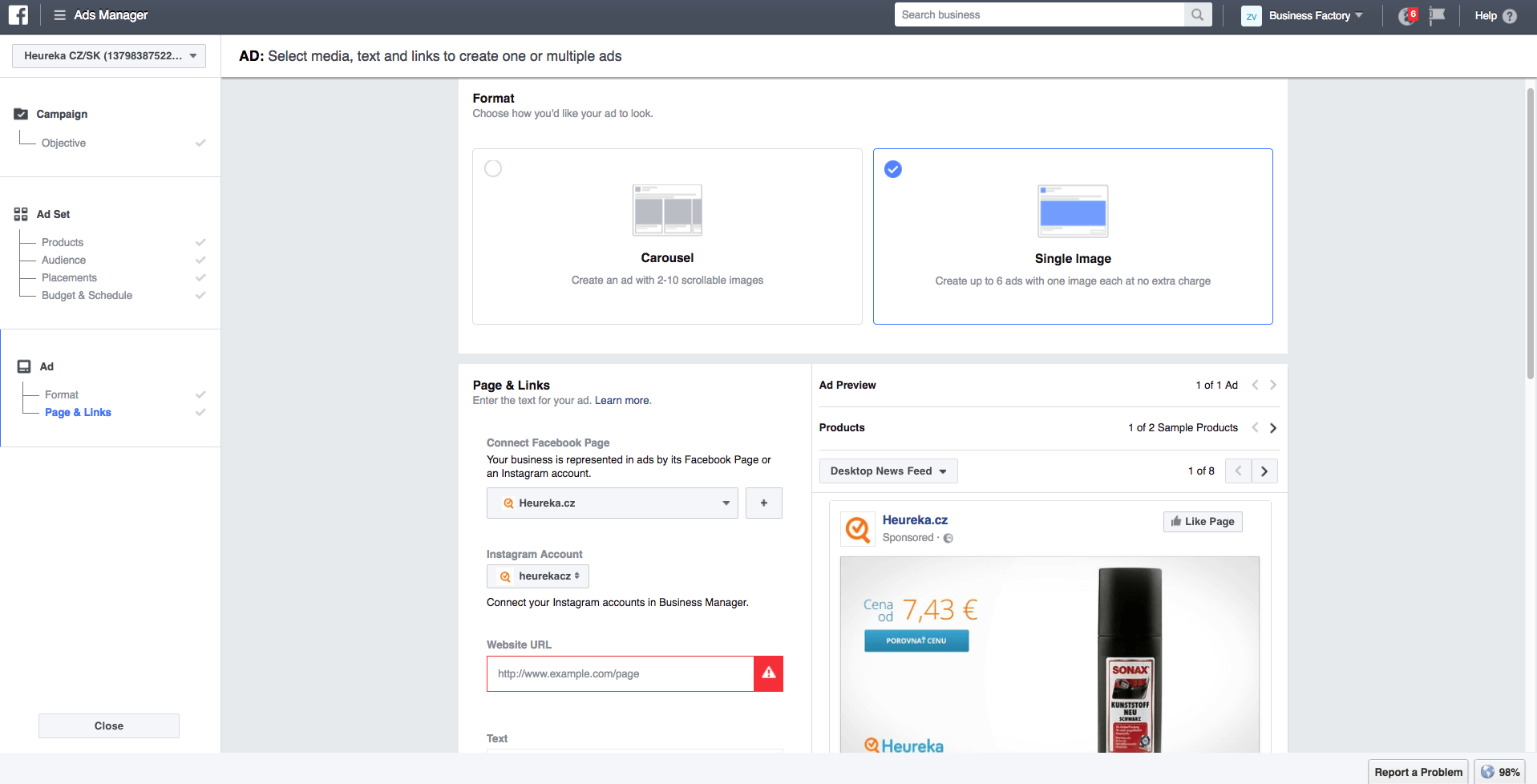This detailed caption provides a thorough description of the Facebook Ads Manager page as seen in the screenshot:

---

The screenshot is of the Facebook Ads Manager utility page, identifiable by the dark gray border at the top and the "Ads Manager" label on the left side. In the upper-left corner, there is a white square featuring a lowercase "f" icon, symbolizing Facebook. Below this icon, the user's account name is displayed, followed by "CZSK" and a long numerical sequence in parentheses.

The left sidebar has a white background and contains three main headers: "Campaign," "Ad Set," and "Ad." The center of the page dominates the view with a large white section. At the top of this section, labeled "Format," users are prompted to choose their ad's appearance. Two options are available: "Carousel" on the left, which allows multiple images to be scrolled through, and "Single Image" on the right, which is the selected option in the screenshot.

Below the format selection, more detailed ad configuration settings are visible, along with a preview of the user's ad. The preview shows a partially visible bottle with a black cap and a white label. The label appears to read "SOMAX" in red letters. Also on the label, there is a small, illegible red square. On the left side of the preview, the company name "HEUREKA" is written in light blue. The company logo, an orange circle with a check mark, accompanies the name.

---

This detailed caption provides a clear and comprehensive description of the Facebook Ads Manager page as depicted in the screenshot.